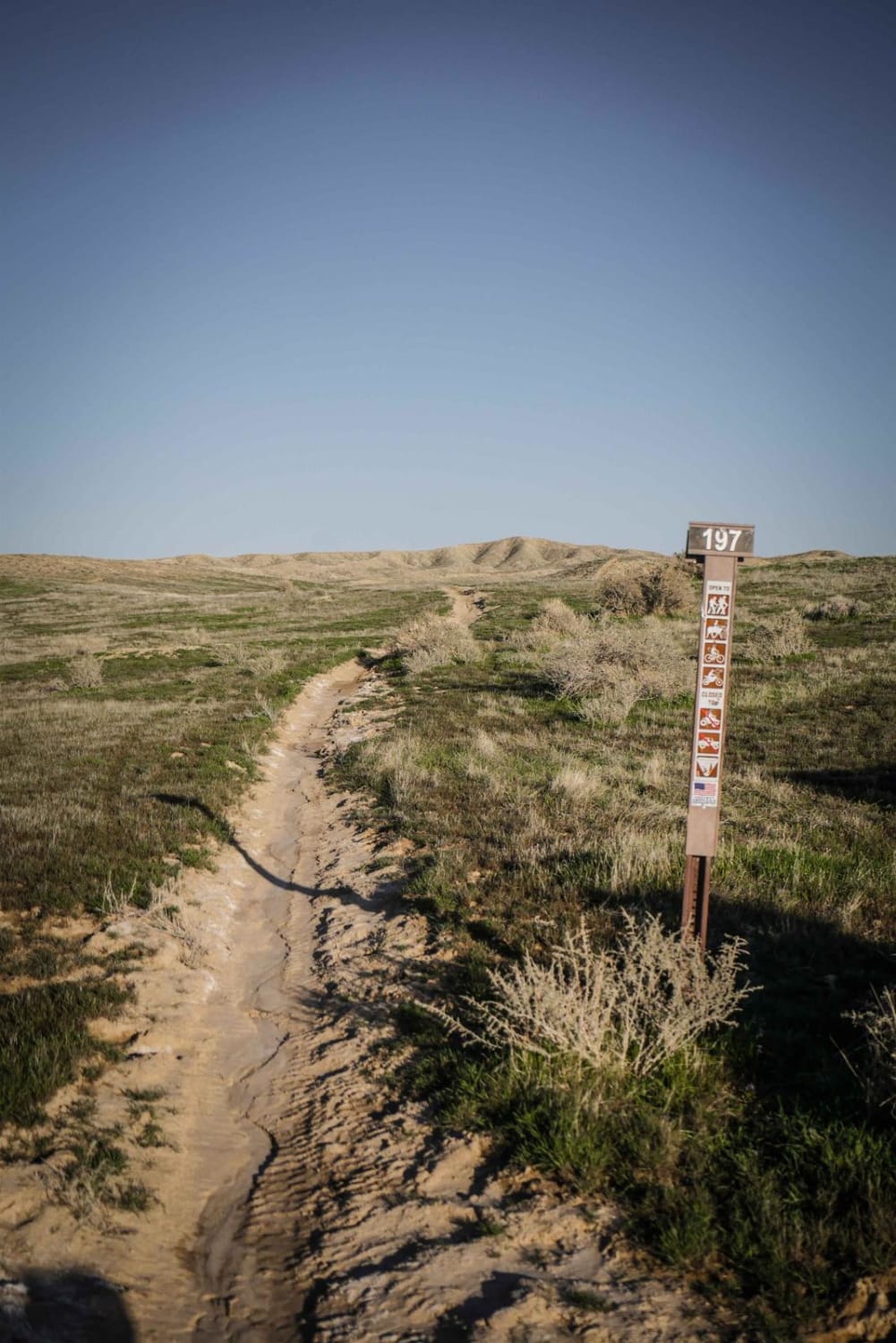This detailed caption follows:

The photo showcases a narrow, sandy trail cutting through scrubland and leading toward low, brown-colored hills in the background, all beneath a clear, cloudless blue sky. This well-worn path features visible bike or motorcycle tracks indicating frequent use, and is surrounded by low-growing vegetation and brown shrubbery that lacks greenery. On the right side of the trail stands a pole with a small sign attached, featuring the number "197" at the top. Below the number, the sign displays pictographs indicating the trail's permissible activities, which include hiking, horseback riding, biking, and possibly motorcycling, though motorcycles are potentially prohibited. An American flag symbol is depicted at the bottom of the sign. The scene is brightly lit by the sun, which casts shadows onto the trail and the surrounding vegetation. Overall, the trail gives an impression of a quiet, yet well-used path through a semi-arid landscape.